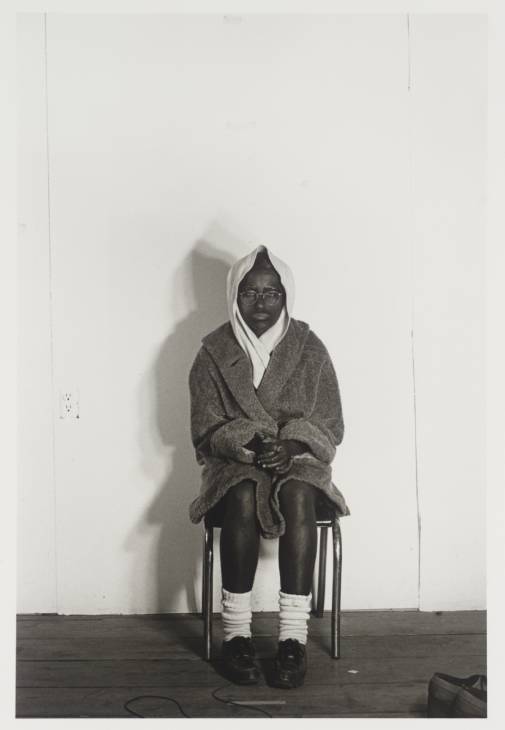The image is a black and white photograph of a solitary African-American man seated on a wooden chair in a sparse room. The room has a stark white background and a floor covered with dark wooden planks. The man is dressed in a dark-colored robe that reaches his knees, with a white hood or scarf covering his head, white socks, and black shoes. His legs are bare below the robe. He sits with his hands clasped together in his lap and his eyes closed, conveying an air of sadness or loneliness. The man wears glasses, and his face is marked by a contemplative expression. A shadow is cast on the wall behind him, enhancing the feeling of solitude. There is a cord stretched across the floor beneath one of his feet, running towards the photographer or viewer, and the edge of what appears to be a handbag is visible in the bottom right corner of the image. An outlet on the wall is also discernible to his right. The overall composition underscores a theme of isolation, captured poignantly in monochrome.